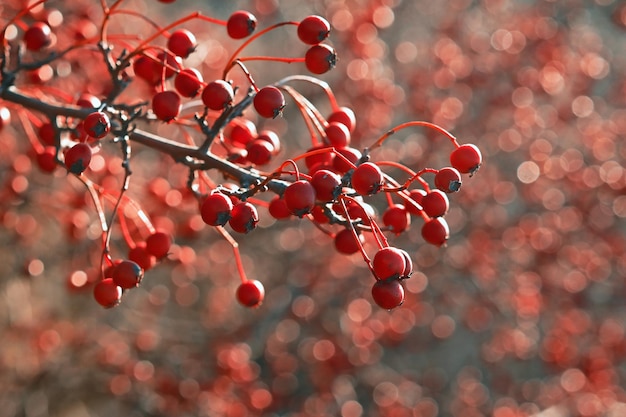The image showcases a detailed close-up of a tree branch adorned with clusters of small, dark red berries. The branch, which is a dark grayish-brown, extends from the left side of the frame towards the center. Each berry is attached to vibrant red stems and features dark spots at their bases. The berries appear heavy, causing the stems to arch downward. In the background, which is blurred to emphasize the foreground, there are more out-of-focus red and pink dots, likely additional berries, along with occasional white spots and gray swirls. The photograph captures a rich contrast between the in-focus foreground branch and the dreamy, indistinct background, highlighting the intricate details and color variations of the berries and the branch.